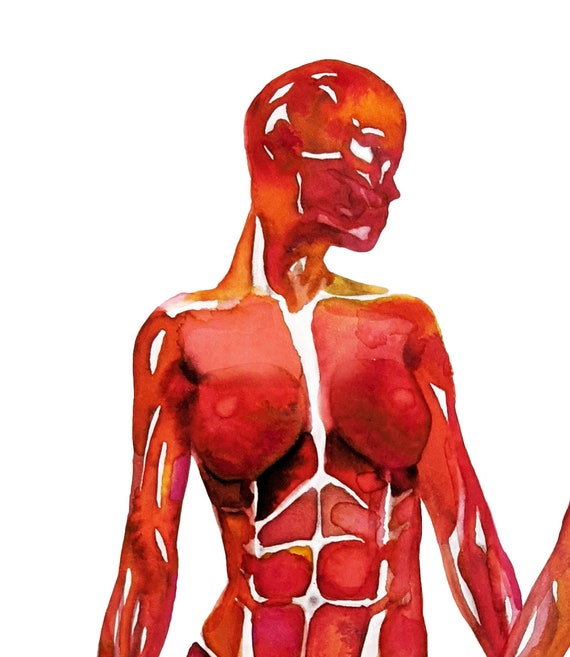This highly stylized drawing depicts a woman's body in a dark, almost skeletal form, primarily using a deep red color palette to mimic the musculature beneath the skin. The image, cut off just below the belly button, showcases intricate detailing with accents of orange and yellow, particularly around the forehead and neck, transitioning into a tan-orange on the shoulders. Her face is turned to the side, with no hair, and features white detailing above the ears, along the cheekbone, and dripping from the nose, giving a slightly surreal effect. The eye is rendered white, adding to the haunting depiction. The white paint also delineates the muscles and separates them, emphasizing the abdomen with visible layers of muscle and the chest area with a stark white line down the breastbone. The arms are positioned down, with partial visibility and a suggestion of another arm cutting off ambiguously. The overall feel is that of a human form painted to expose the underlying anatomy in a visually striking and artistically exaggerated manner.